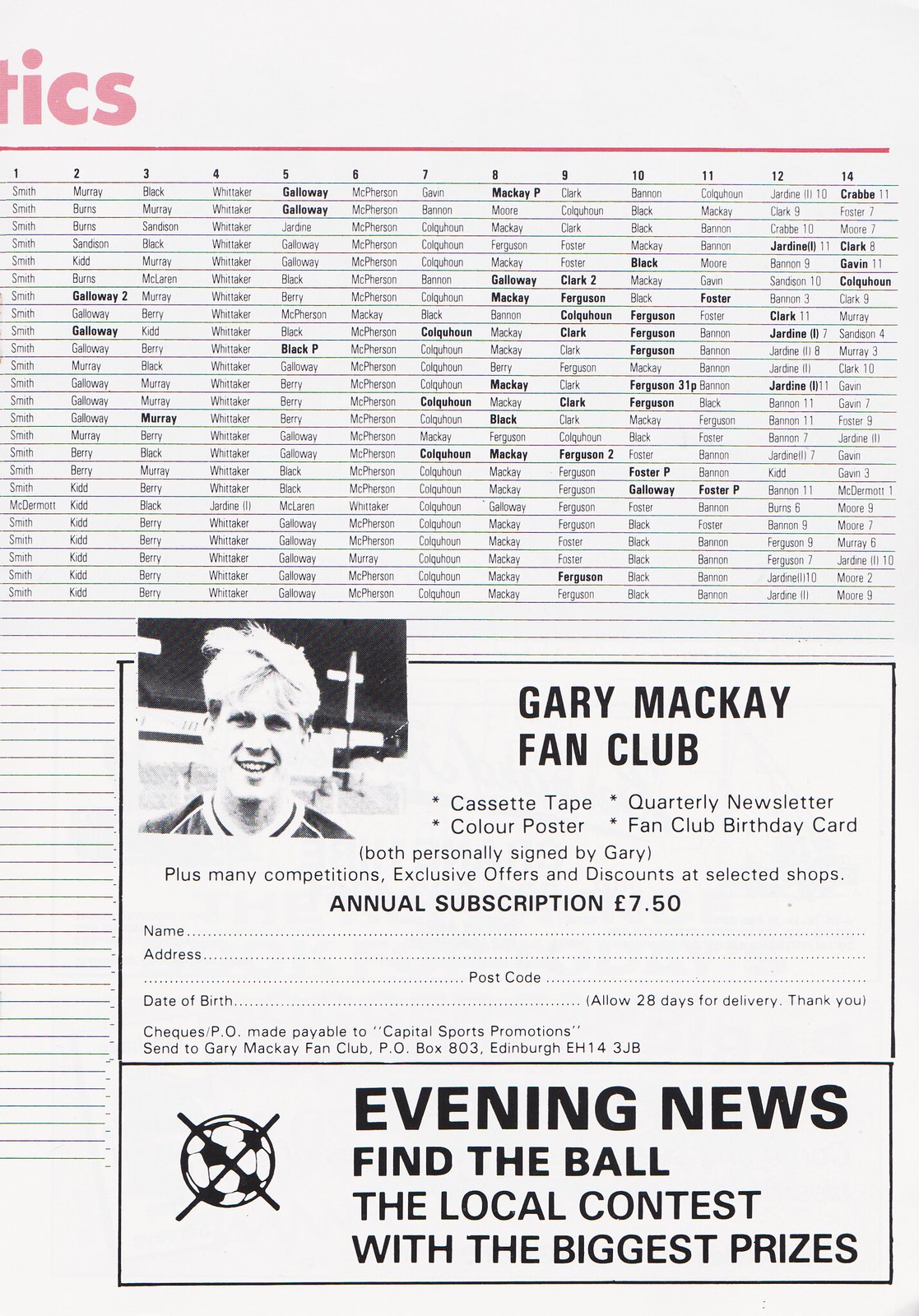The page, likely taken from a football program or a similar publication, is taller than it is wide and predominantly black-and-white with selective red highlights. At the top left, the red lettering "TICS" and a red horizontal pinstripe span the page. Below this pinstripe is a grid formed by black pinstripes, with the numbers 1 through 14 running horizontally across the top, followed by rows of player last names. This table, possibly showing rankings, placements, or player information, continues from a previous page.

The bottom half of the page features two rectangular segments. The upper segment promotes the Gary McKay Fan Club, including a photograph of Gary McKay, a smiling Caucasian man with light, messy hair. Details of the fan club perks are provided: a cassette tape, a quarterly newsletter, a color poster, and a personally signed fan club birthday card, along with competitions, exclusive offers, and discounts. Membership costs £7.50 per year. There’s a form for personal details and instructions to allow 28 days for delivery, with payment made to Capital Sports Promotions and mailed to Gary McKay Fan Club, P.O. Box 803, Edinburgh, EH143JB.

Below this, an advertisement for the "Evening News Find the Ball" contest claims it offers the local contest with the biggest prizes and shows an image of a soccer ball with an X through it.